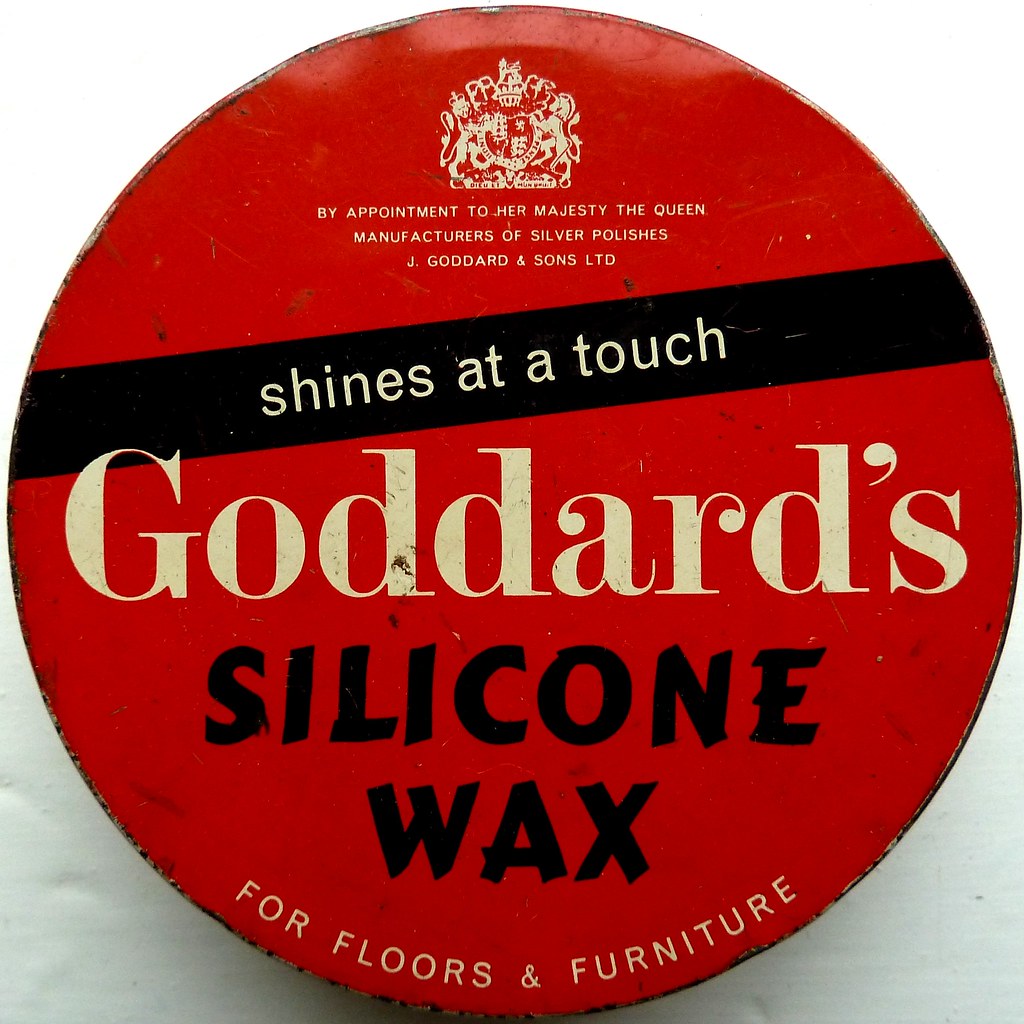The image is a close-up of an old, round, red metallic-looking lid, centered in the frame. At the top, there's a crest featuring two lions and a crown. Beneath this crest, in small white letters, it reads, "By Appointment to Her Majesty the Queen, Manufacturers of Silver Polishes, J. Goddard & Sons Ltd." A black diagonal stripe crosses the lid with the phrase "Shines at a Touch" in white letters. Prominently displayed in large white font below the stripe is the brand name "Goddard." Beneath this, in black font, it says "Silicone Wax." Encircling the bottom edge of the lid, in white letters, is the text "For Floors and Furniture." The colors on the lid are mainly red, black, and white, with some of the text appearing slightly yellowed, likely due to the age of the packaging.